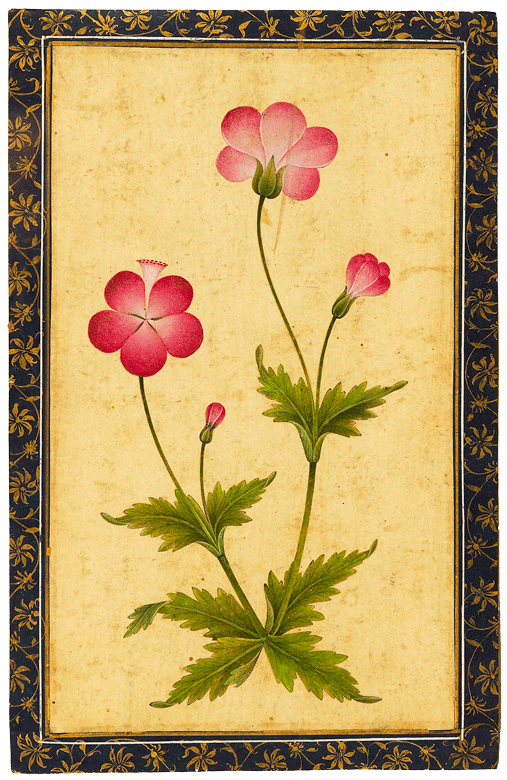This artwork illustration features a vibrant depiction of a flowering plant set against a tan and dark splattered pattern background that mimics an aged paper look. The plant consists of two main green stems sprouting from a base with four green leaves. Each stem supports two blooms, totaling four flowers. The two larger flowers, illustrated in a striking red-pink hue with some white accents, are the most prominent. The left stem bears one large flower with about five petals and a smaller budding flower, while the right stem mirrors this arrangement but with the smaller bud beginning to open. One of the flowers features a distinctive nectar pod poking out from its center. The tallest flower sits at the top, crowning the composition. The artwork is framed by a border of black with intricate gold flower and vine designs, adding an ornate touch to the piece.